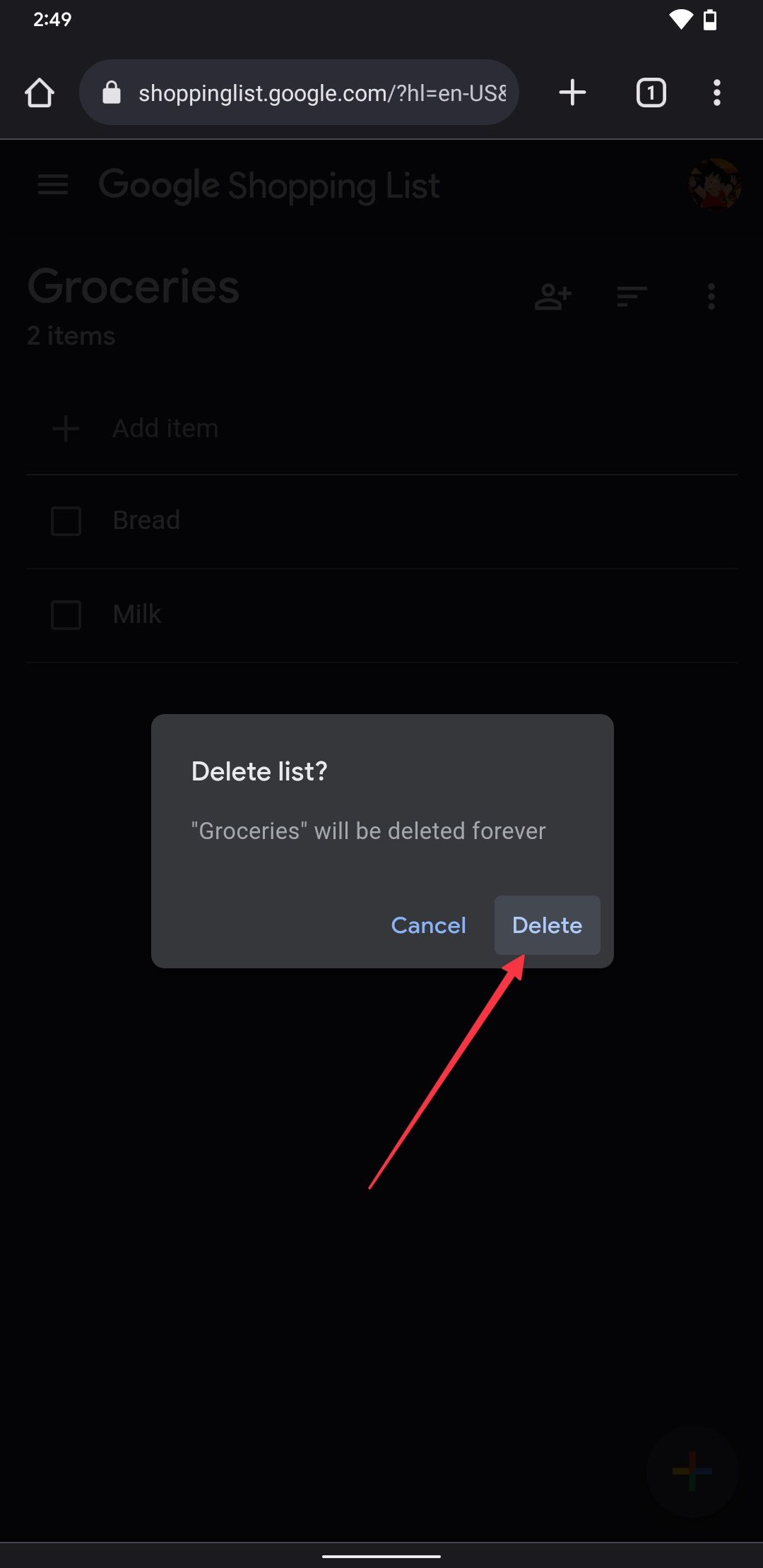An individual has searched for "shoppinglist.google.com" on their phone, navigating to the shopping list page. The screen shows a minimalistic layout featuring a home button on the left and a plus sign on the right, with an additional tab indicator labeled "1" and a settings menu represented by three vertical dots.

The upper section of the webpage prominently displays "Google Shopping List," but this heading is partially faded due to an active dialog box that has appeared at the bottom. This gray dialog box asks whether the user wishes to delete the "Groceries" list permanently, with a red arrow pointing upwards to the "Delete" button. The dialog box also includes a "Cancel" option, both in blue text.

In the main content area, which has a black background, the page title "Google Shopping List" is followed by three lines on the left and the option to add an account on the right. The subtitle "Groceries" is displayed prominently with user controls nearby. Below, it notes that there are two items on the list with options to add an item or mark items as completed. Each list item, such as "Bread," is accompanied by a checkbox for user interaction.